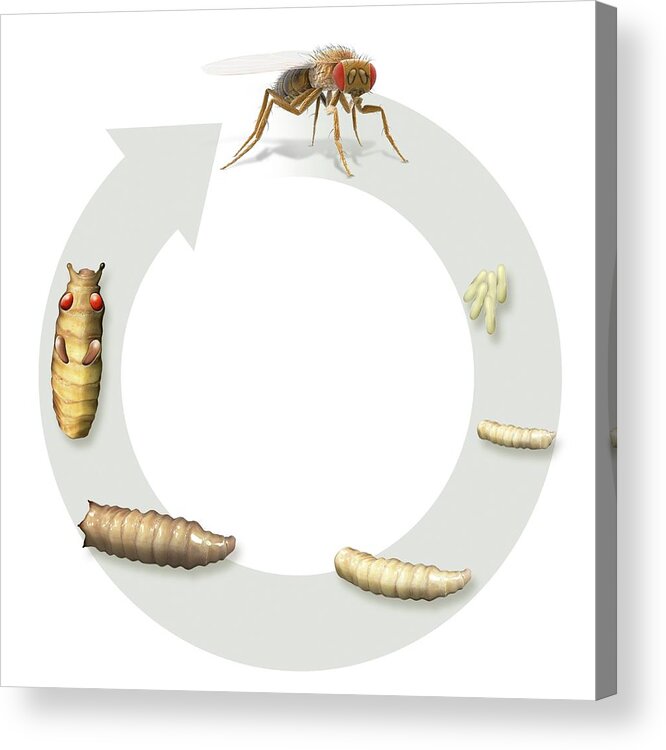This color illustration diagram, set against a white background, intricately depicts the life cycle of a fly. At the top of this circular diagram is a detailed brown housefly, oriented to the right. The fly sits atop a light gray circular arrow that loops clockwise, illustrating the progression of stages. Below the fly, in sequential order, are four white eggs, followed by images of increasingly larger maggots. The final maggot, distinctly detailed, features bright red eyes, small antennae, and visible appendages, representing the stages of metamorphosis before returning back to the fly at the top. The image is void of text and employs a muted brown and white color scheme, crafted on a white canvas that accentuates the cycle's flow and detail.